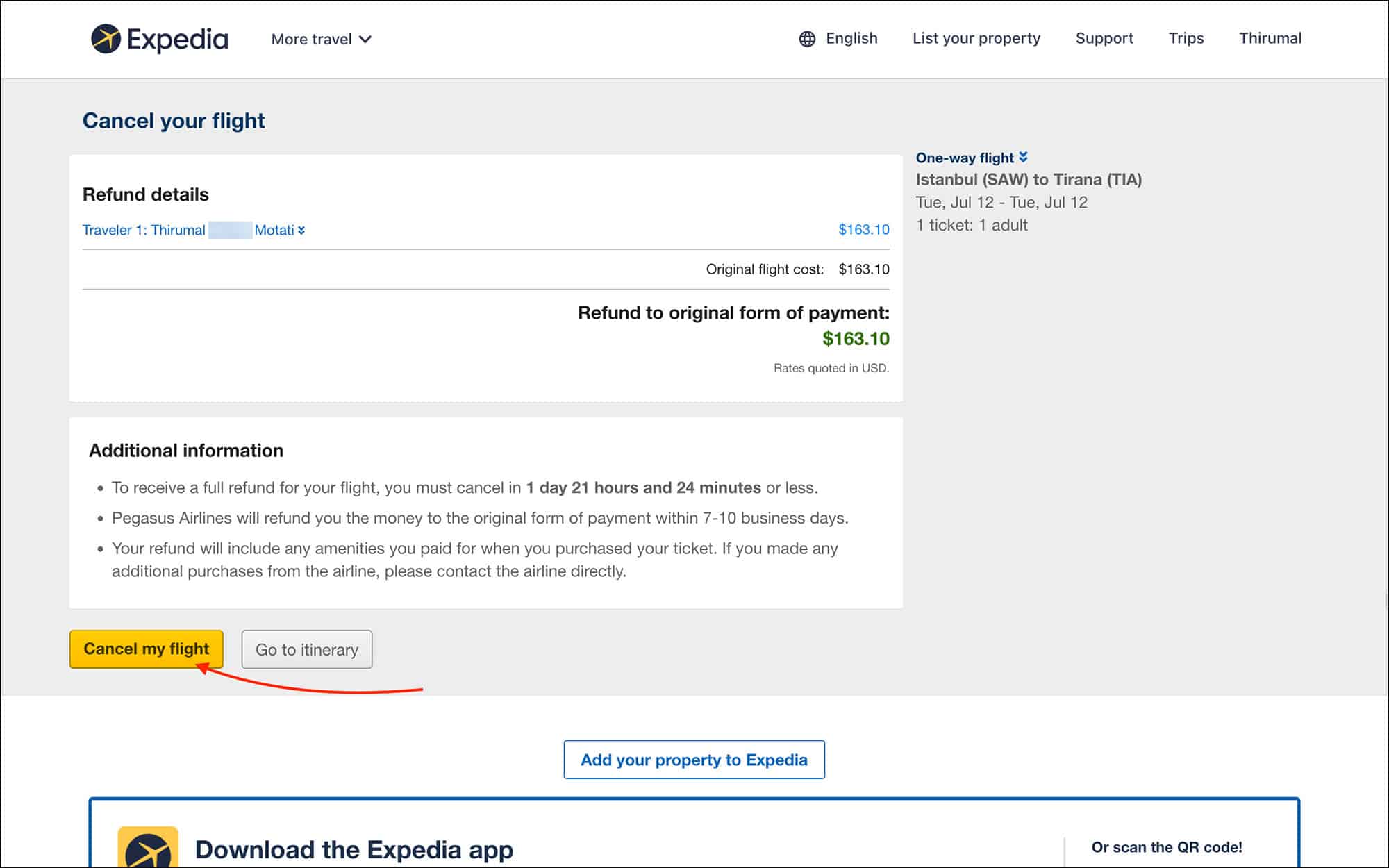The image is a screenshot from the Expedia website. At the top, there is a white bar with the Expedia logo on the left, which includes a yellow airplane inside a circle. To the right of the logo, there is a dropdown menu labeled "More Travel," followed by several options: "English," "List your property," "Support," "Trips," and a UML navigation link.

The middle section features a gray background with a blue heading on the upper left that reads "Cancel your flight." Below this heading, there are two prominent white rectangles.

The first rectangle displays refund details:
- It lists the traveler's name: "Thermal Moti."
- The price is shown as $163.10 with the following breakdown: the original flight cost is $163.10, and the refund to the original form of payment is also $163.10. The rates are quoted in USD.
- To the right, it details the flight information: a one-way flight from Istanbul (SAW) to Tirana (TIA) on Tuesday, July 12th, for one adult.

The second rectangle provides additional information:
- It states that to receive a full refund, the flight must be canceled within 1 day, 21 hours, and 24 minutes or less.
- Pegasus Airlines will issue the refund to the original form of payment within seven to ten business days, which includes any amenities purchased with the ticket.
- It advises contacting the airline directly for additional purchases made from the airline.

At the bottom left of the image, there is a yellow button labeled "Cancel my flight" with a red arrow pointing to it.